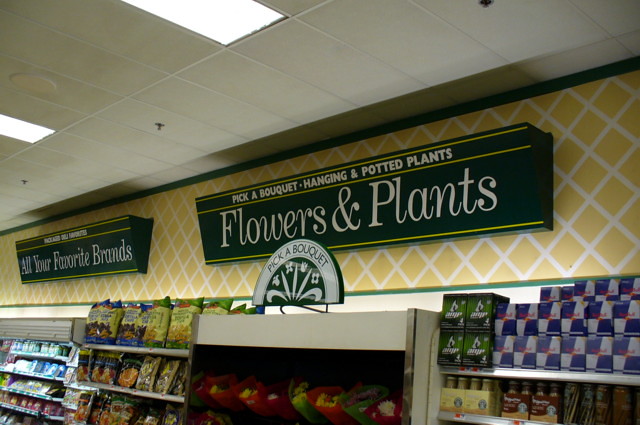The photograph captures the interior of a convenience store. Prominently featured in the center is a display of fresh, cut flowers dimly lit within a case, topped with a sign that reads "Pick a Bouquet," echoing the message of another sign hanging above amidst potted plants and flowers. To the left of the floral display, a rack of snack chips, organized in bags on shelves, presents a variety of quick bites. Further left, a cooler stocked with assorted products extends the array of available items. In the foreground on the right, two shelves are filled with beverages, notably including Red Bull energy drinks, green cartons, and multi-packs of bottled drinks. The top of the wall and ceiling frame the scene, adding to the cozy, bustling atmosphere of this well-stocked convenience store.